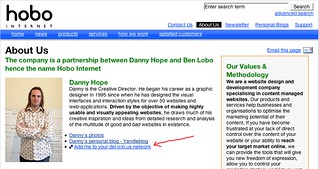In the upper left corner of the image, in black text, are the letters "H-O-B-O," with "Internet" in very small text underneath. To the right, there's a search bar followed by a long blue bar underneath it, with the text "About Us" in black. 

The company, named Hobo Internet, is a partnership between Danny Hope and Ben Lobo. Their namesake is displayed in green text with "Danny Hope" specifically highlighted in green. To the left of this text, there is an image of Danny Hope. He has shoulder-length brown hair and is wearing a long-sleeved, white-collared shirt with a print on it. The background wall behind him is beige at the top and white at the bottom, and he has his hands crossed against his chest.

To the right of Danny's image, there is a clickable area labeled "Danny's Process" in blue, underlined. Next to this, there is another blue text area with a red arrow pointing to the right. Further to the right, in green text, it says "Our Values and Methodology," followed by a long informational paragraph underneath.